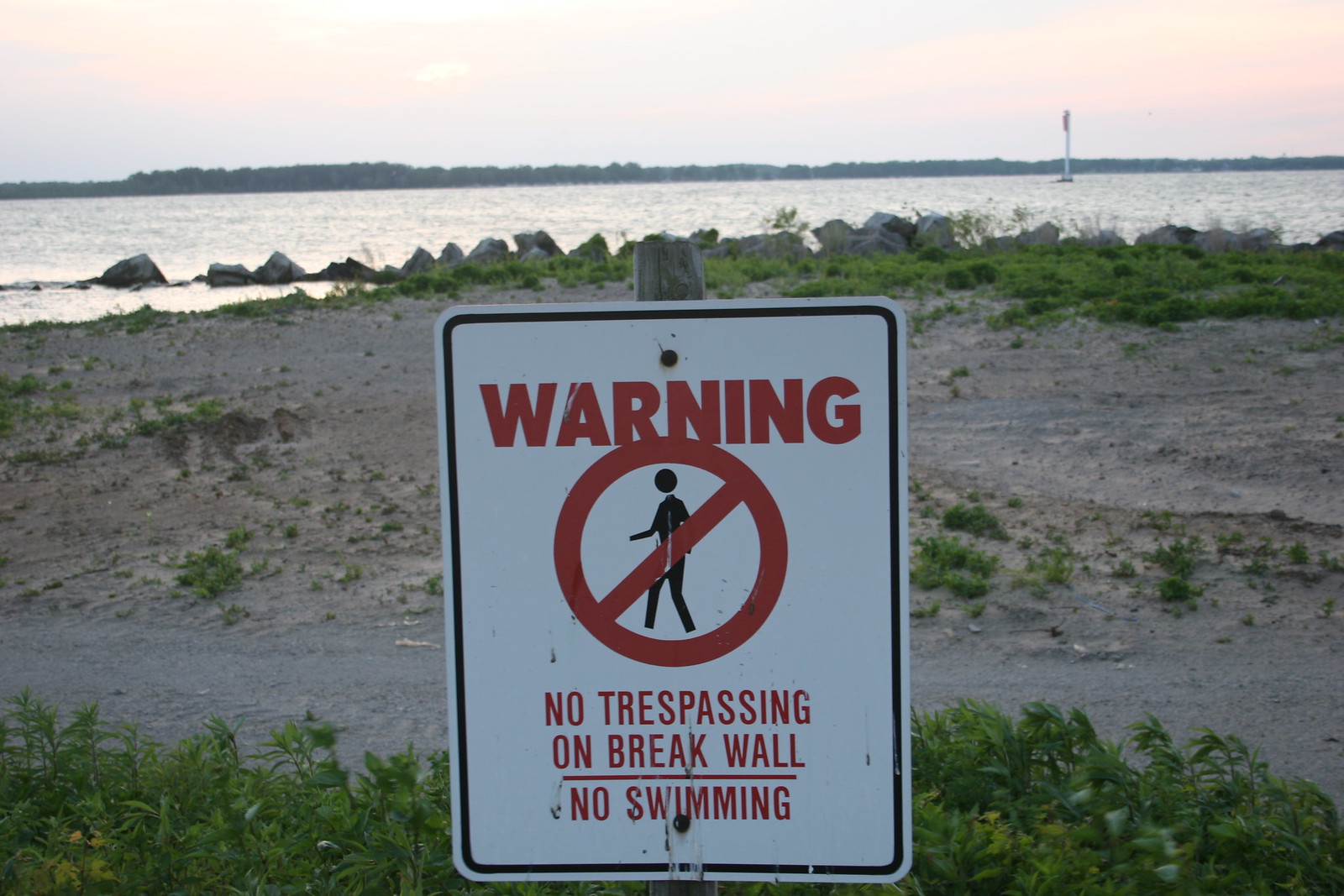The photograph depicts a serene late afternoon or early evening setting at a beach. The image is a horizontal rectangle with the horizon line positioned towards the top. Above the horizon, the sky is tinged with a hazy peach color, suggesting the onset of dusk. Beneath the horizon, there is a calm expanse of water which meets a break wall composed of rocks. 

Central to the bottom of the image, there is a clearly visible sign. The sign has a white background with red and black text that reads "WARNING: No Trespassing on Break Wall, No Swimming." It also includes an illustration of a person with a red prohibition sign over it. Surrounding the sign is a combination of natural colors: green from the scattered foliage, beige and black from the beach sands and rocks, and various shades of gray. The overall ambiance conveyed by the photograph is peaceful yet cautionary, capturing the tranquil beauty of the beach juxtaposed with the warning sign's stern message.